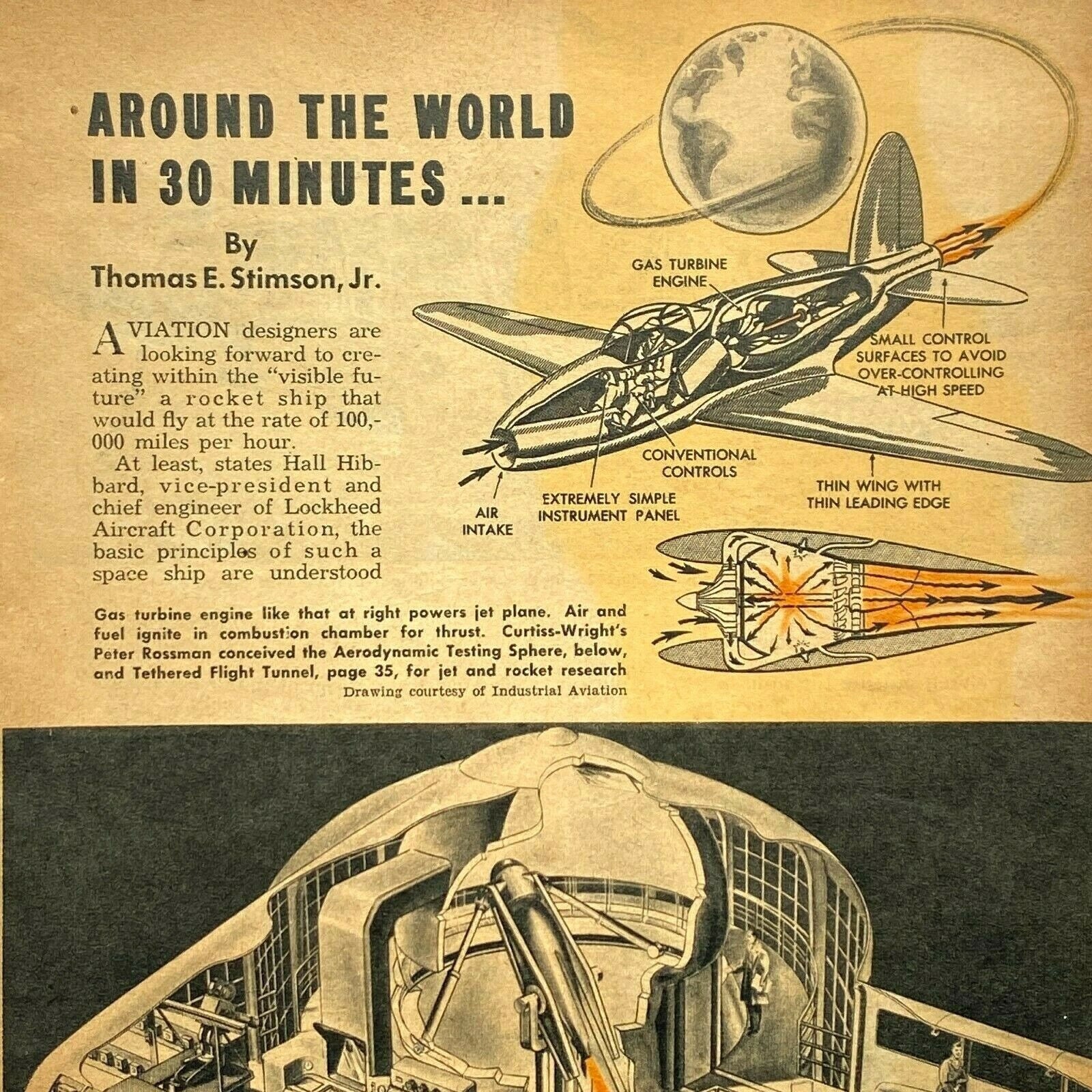This image features a full-page article from an aged aviation or scientific journal, evident from the yellowed paper and dated typographic style. The article, titled "Around the World in 30 Minutes" by Thomas E. Stimson Jr., explores the concept of a high-powered jet capable of circumnavigating the globe at speeds reaching 100,000 miles per hour. Detailed illustrations accompany the text, including a cross-section of a single-engine gas turbine aircraft, showing the pilot’s position and the mechanics of the engine. Another diagram provides a close-up of the jet engine's inner workings, while a third image depicts what appears to be a viewing area or launch pad for the aircraft. The article’s ambitious vision reflects a bygone era’s fascination with rapid global travel through advanced jet propulsion technology.